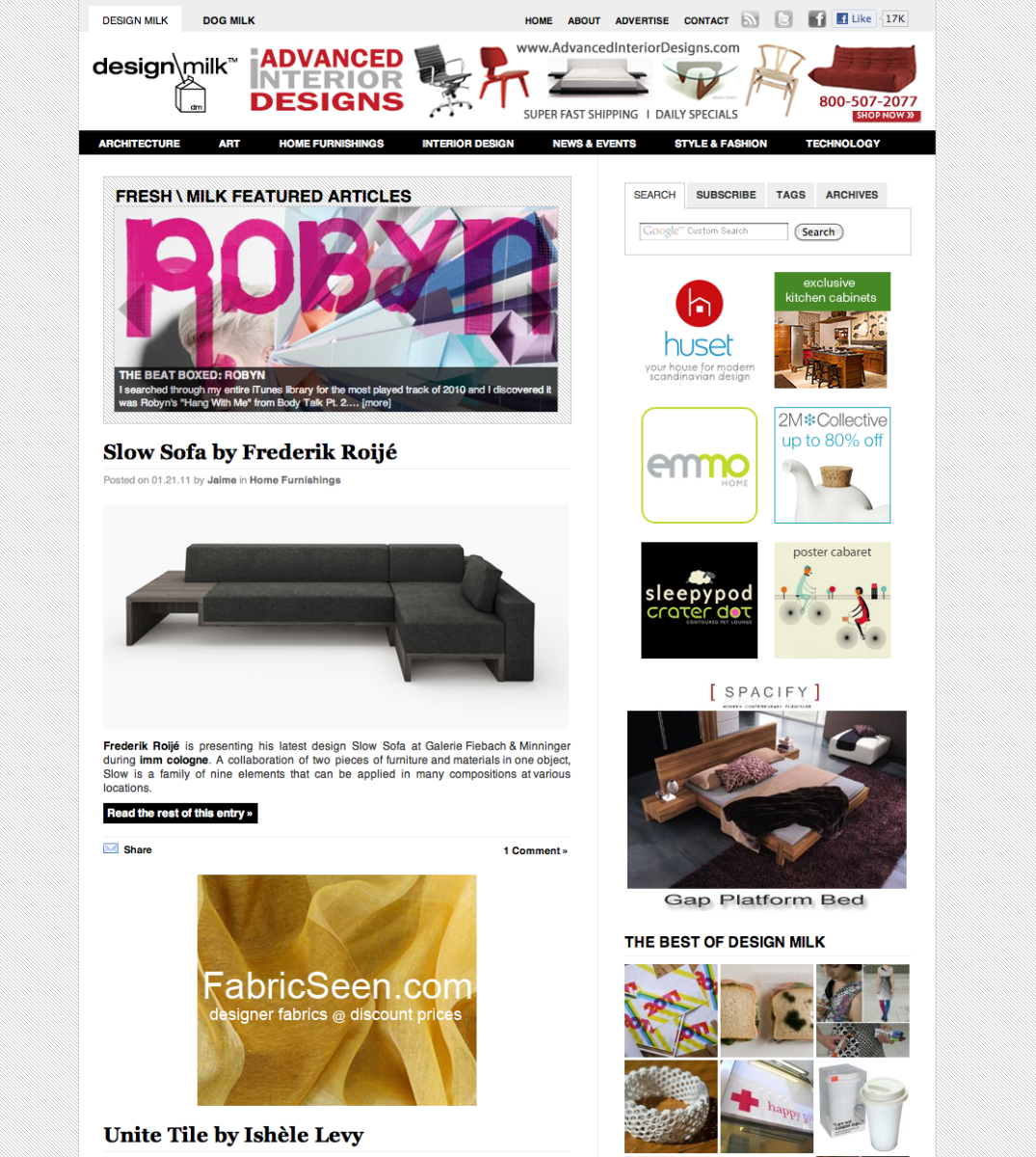The image displays a webpage with the title "Design Milk" prominently featured at the top, followed by a section labeled "Dog Milk." Below these titles, the navigation menu includes options such as Home, About, Advertise, and Contact. 

The central area showcases various elements arranged in square sections. One square highlights the Facebook icon with a "17K" like count. Another section is titled "Design Milk Advanced Interior Designs" in red and gray font and features images of two chairs, one black and one red. 

Adjacent to these chairs is a promotional link to the website www.advancedinteriordesign.com. Further down, there are images of a bed, a table, a beige chair, and a red couch. Beneath this is a call to action with the contact number 800-507-2077 and a "Shop Now" button.

The section titled "Fresh Milk Featured Articles" includes a highlight of an article named "Robin the Beatbox Robin." Below this article is an image of a couch known as the "Slow Sofa" by Frederick Rogge, accompanied by a section for sharing and commenting.

Moreover, there is a mention of "Fabricscene.com: Design of Designer Fabrics at Discount Prices" and an introduction to "Unite Tile" by Assaf Levy. To the right of these elements, the page showcases various brands and products, such as the "Hush Set Emo," "Sleepy Pod," "Crotter," "Spacify," and "Gap Platform Bed," indicating a curated selection under "The Best of Design Milk."